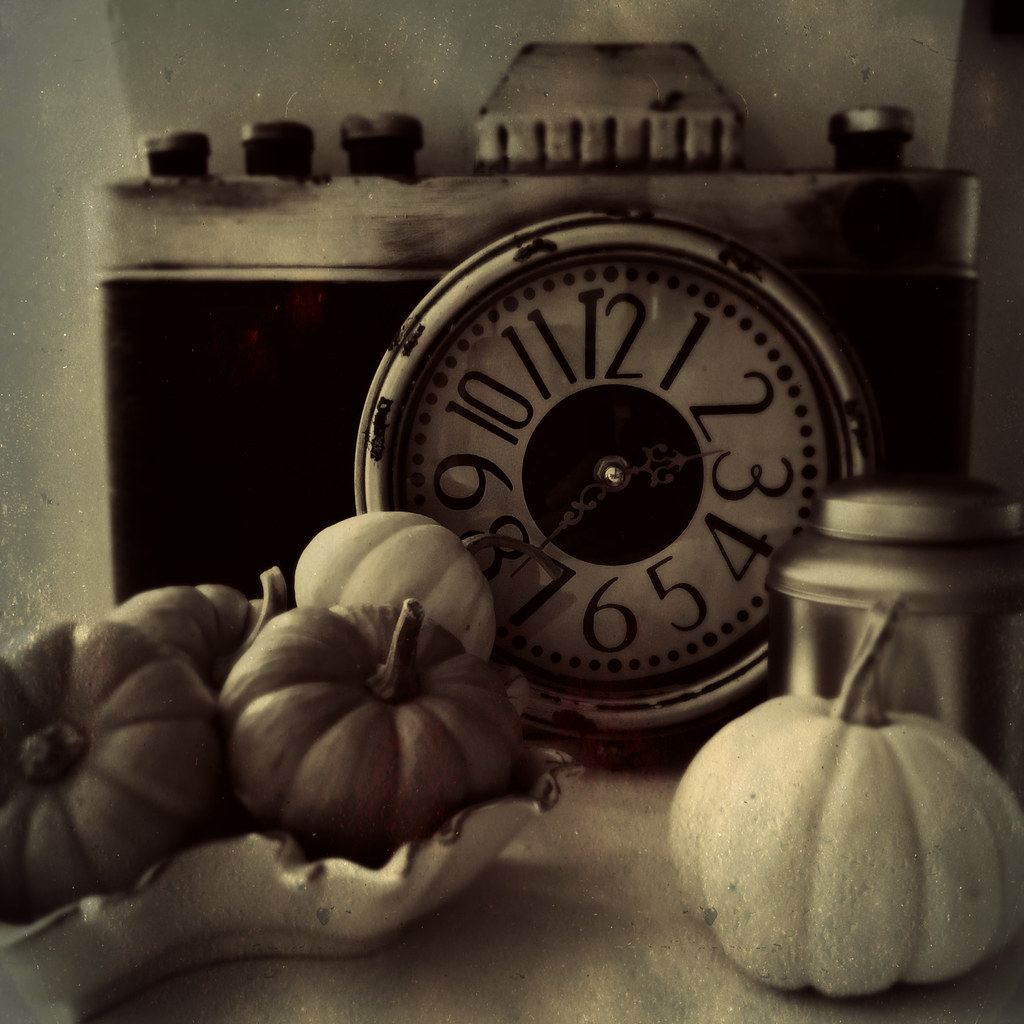This vintage-style photograph, characterized by its black, white, grayscale, and sepia tones, captures a quaint still-life scene. On the left, a curved ceramic dish holds four small gourds—three resembling dark-colored pumpkins and one in white. Dominating the right side of the image is a larger white pumpkin or gourd. Behind this arrangement, a jar with a metal lid sits unobtrusively. The background is dominated by a large, retro camera-like device that resembles a clock. This clock has a round dial featuring numbers 1 through 12 and hands, suggesting it is indeed a functioning timepiece. The clock's rectangular body is topped with a horizontal metal band and adorned with four buttons, adding to the vintage aesthetic.